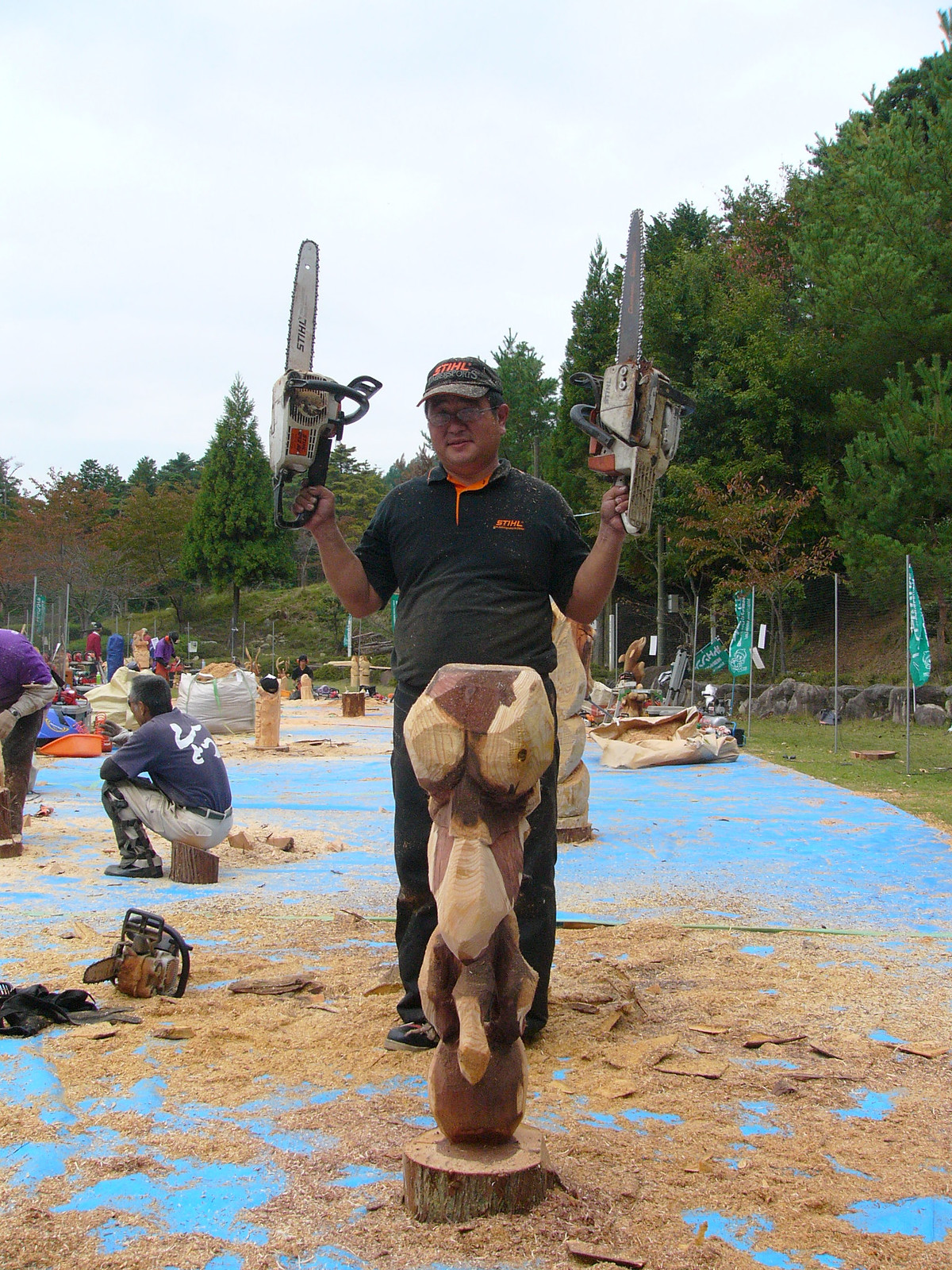This detailed image depicts an outdoor wood sculpture competition set on a green field with sawdust scattered on a light bluish tarp. At the center stands an Asian man proudly holding two white steel chainsaws with black handles—one in each hand—raised high. He wears a gray shirt and pants, black boots, and a brown baseball cap featuring the orange "Steel" logo, which matches the branding on his shirt. The man is also wearing glasses. In front of him is a wooden sculpture, appearing to depict a monkey with light sections around its eyes, nose, and arms, standing amidst sawdust. To his left, another chainsaw lies on the tarp. Seated nearby on a log is a gentleman in a blue shirt and gray pants, engaged in woodwork. The backdrop features several other participants working on various wooden sculptures, surrounded by green trees, grass, and green vertical banners with white lettering indicating a chainsaw contest. The scene is accented with the colors of autumn, as some of the trees display reddish hues.